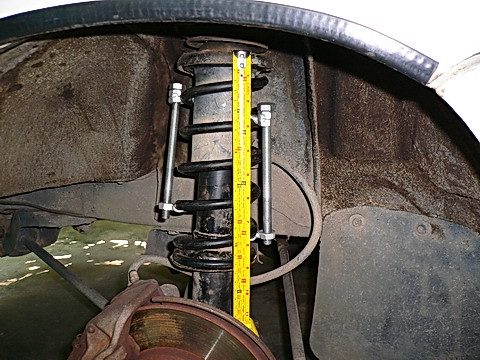In this detailed image, we observe the intricate components of a car's wheel axle assembly, prominently featuring the suspension and brake system. The focal point is a black suspension spring positioned centrally, with a yellow tape measure running alongside it. The background is predominantly white, curving towards the top, possibly indicating an indoor setting. The bottom right of the image displays a rusted metal brake disc, partially cropped off, suggesting the wheel and rim are absent. Surrounding these elements are various bolts, metal struts, and a metallic plate, complemented by the vivid colors of gray, brown, black, red, green, tan, and yellow. The spring appears sizable, indicating a large vehicle. No text is visible throughout the image. The overall scene gives the impression of an exposed brake and suspension system, possibly from the underside of a car.